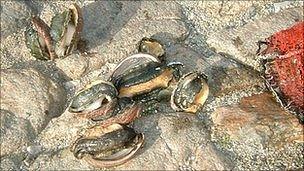The image depicts a coastal scene with a rocky or cobbled surface, possibly along a beach or seaside. In the center, there are several dark-colored mussel shells, some showing an orange fleshy interior. Specifically, four shells are clustered together in the middle, while two more sit side-by-side in the upper left corner, casting shadows on the ground. An additional single shell is located at the bottom center of the image. The rocks in the background display various textures, and the lighting suggests it is daytime, with bright sunlight creating stark contrasts. On the right edge, there is a red, textured object with frayed edges, possibly a piece of fabric or a fisherman's net, contributing to the coastal atmosphere of the scene. The water has darkened some of the rocks near this red object. Overall, the colors in the image range from the bright sunlight illuminating the scene to the darker tones of the shells and rocky surface.